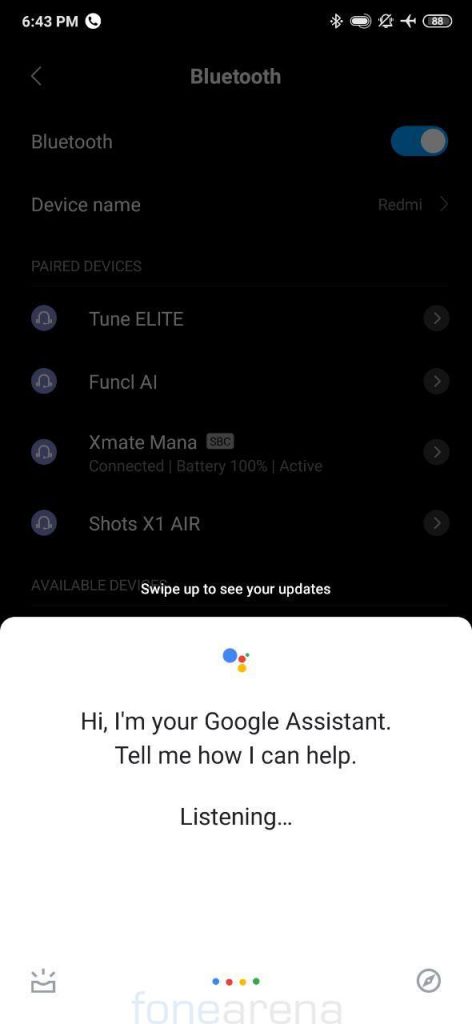The vertically rectangular image appears to be a screenshot from a smartphone. The upper portion of the screen is shadowed, displaying the Bluetooth settings section. The Bluetooth toggle is turned on, and it shows a label for the device name, although it is obscured by shading. Below the toggle, a list of available Bluetooth devices is visible. 

At the bottom of the screen is an active pop-up window with a white background. The pop-up is from Google Assistant and contains the text, "Hi, I'm your Google Assistant, tell me how I can help," followed by the word "Listening" accompanied by an ellipsis. 

At the very bottom of the screen, the words "Phone Arena" are displayed in a very light gray color. Centered above this text are the four colored dots representing the Google logo, arranged in blue, red, yellow, and green.